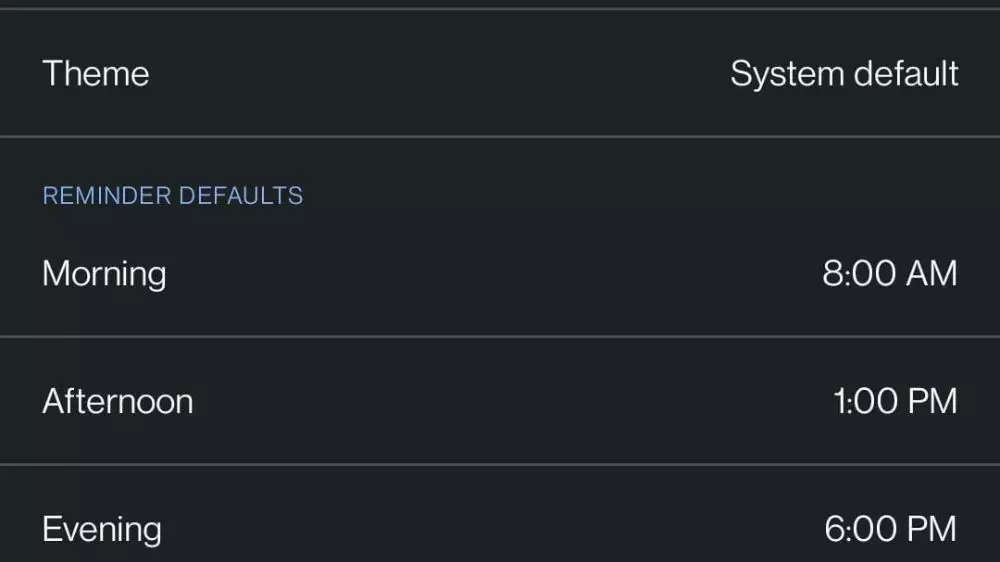A cleaned-up and detailed caption for the image could be:

"A cropped screenshot taken from a phone displaying settings on a black background, featuring four rows with distinct sections. 

In the top row:
- Upper Left: The word 'Theme' is displayed in a light grayish-white text.
- Upper Right: The text 'System Default' appears, with 'System' starting with a capital 'S' followed by lowercase letters, also in the same grayish-white color.
- A horizontal line separates this row from the next.

In the second row:
- Upper Left: The words 'Reminder Defaults' are written in a light bluish-purple uppercase font.
- Below that: The word 'Morning' with a capital 'M' appears in the grayish-white font.
- Upper Right: The time '8 o'clock AM' is displayed. A horizontal line separates this row from the following one.

In the third row:
- Left Side: The word 'Afternoon' is written in the grayish-white font.
- Right Side: The time '1 o'clock PM' is shown. A horizontal line separates this row from the last.

In the bottom row:
- Left Side: The word 'Evening' is displayed.
- Right Side: The time '6 o'clock PM' appears, both in the grayish-white font."